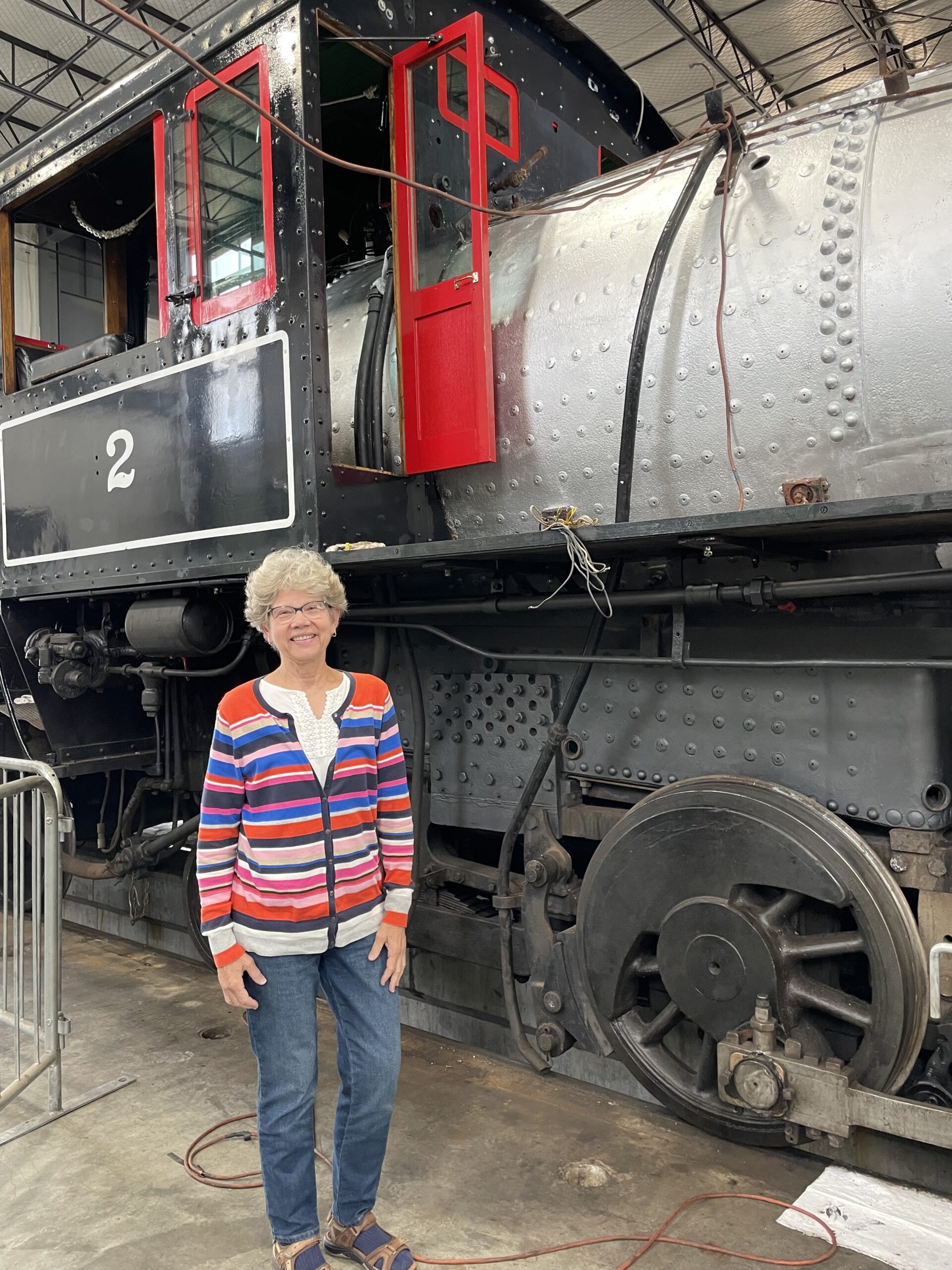In this image taken inside a museum or a rail yard, we see an aged, gray-haired woman wearing glasses, a white shirt, a multicolored cardigan with red, blue, pink, and black horizontal stripes, blue jeans, and Birkenstock sandals. She stands beside a large, classic black steam locomotive, likely from the late 19th or early 20th century. The locomotive features a prominent white number "2" within a rectangular border on its side and has red accenting around the door and sliding window of the operator's cabin. The massive steel wheels rest on a concrete floor, distinguishing the setting as indoors rather than on traditional tracks. The locomotive's steam tank and riveted fuselage add to its historical appearance. The woman stands on the right side of the locomotive, which faces the right side of the image. The connection between the woman and the locomotive remains unclear, adding an element of mystery to the scene.